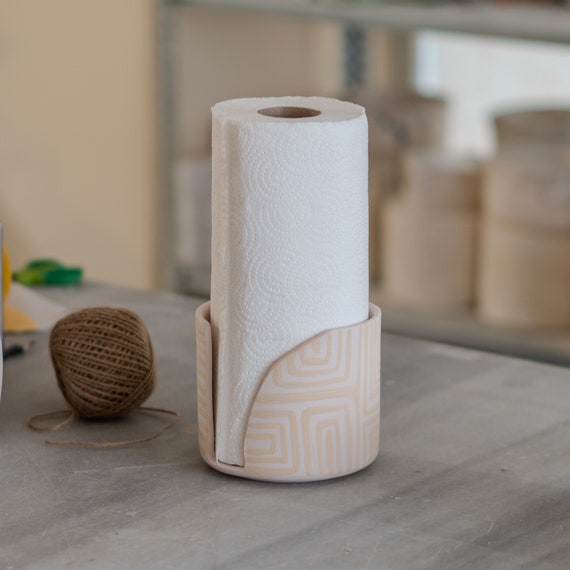The image depicts a unique and contemporary paper towel holder situated on a gray kitchen counter or table. The holder itself is reminiscent of a ceramic cup with a distinctive design; it features a curved cutout on one side and a straight vertical edge on the other. This straight edge can possibly be used to tear off the paper towels. The holder boasts a peach and cream pattern, comprised of interlocking boxes and lines, creating an attractive visual appeal. The roll of white paper towels fits snugly within this holder, which has an open bottom allowing easy access.

Next to the paper towel dispenser lies a dark tan ball of twine, partially unraveled to show a small loop of string that puddles around it. The background, slightly blurred, reveals scissors and shelving that holds round objects like canisters or hat boxes, adding to the kitchen ambiance. A bright green item is also partially visible in the blurred background towards the left, but it remains unidentified. The primary focus remains on the striking paper towel dispenser and the neat roll of paper towels it holds.